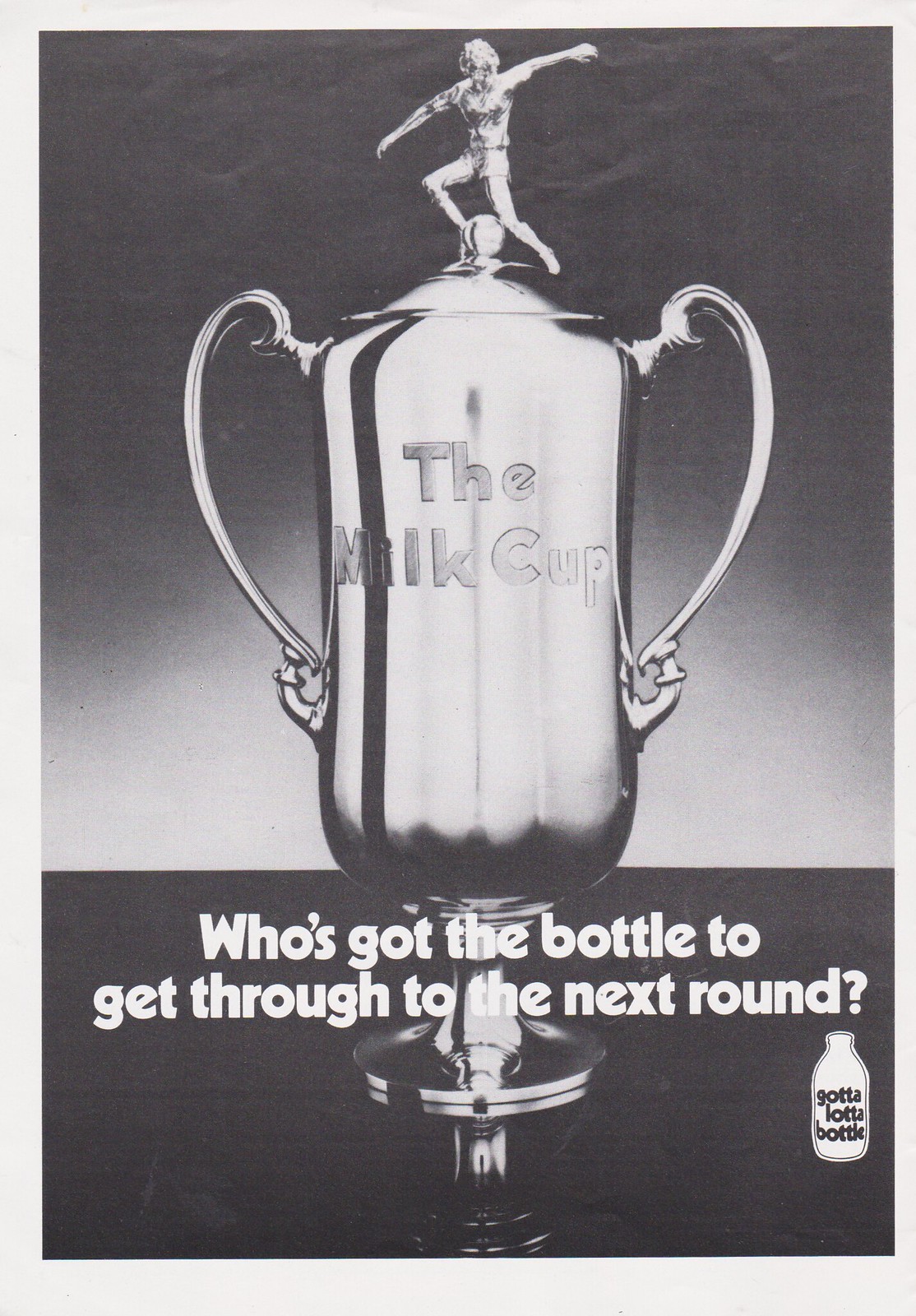This black and white print, likely a vintage magazine advertisement, features a prominent silver trophy at its center, known as "The Milk Cup." The cup is detailed with two ornate, ear-shaped handles extending from its sides and topped with a statue of a soccer player poised with a ball between its legs. This shiny, silver-colored trophy stands out against a gradient background that fades from black at the top to white at the bottom. At the base of the trophy, the phrase "Who's got the bottle to get through the next round" is boldly printed in white text on a black background. In the lower right corner, there is a small white bottle with the phrase "got a lot of bottle" inscribed on it, adding to the thematic consistency of the advertisement. The meticulous composition and nostalgic black-and-white aesthetic suggest an era long past, emphasizing the prestigious nature of the award and the competitive spirit it represents.